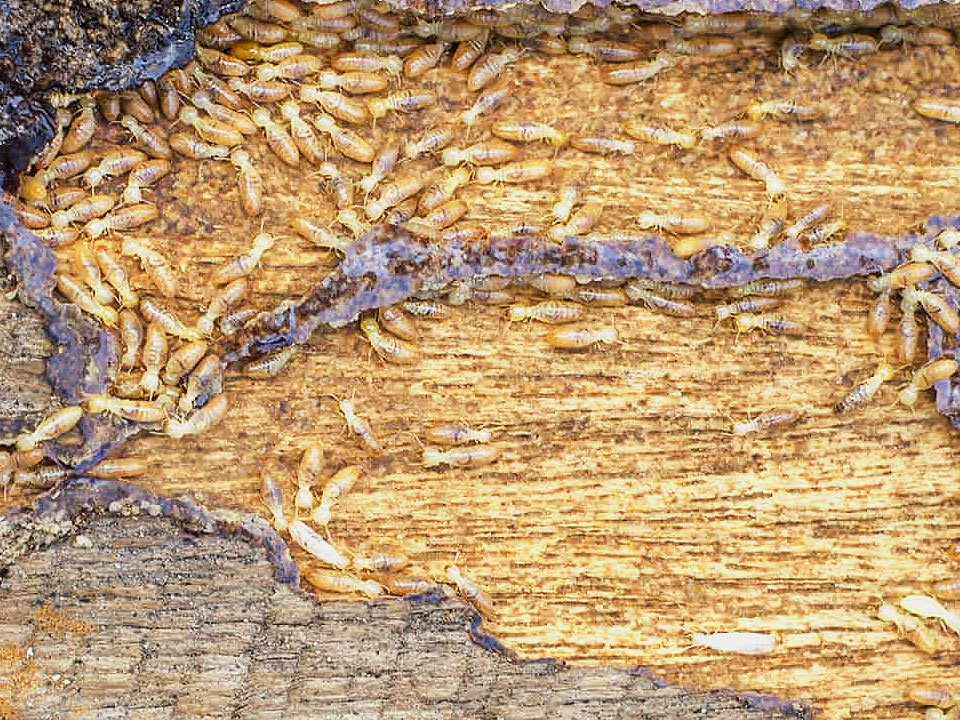The photograph vividly captures a close-up view of numerous termites voraciously consuming a piece of exposed, yellow-grained wood. The wood is barren and bare, with hints of gray bark visible in the lower and upper left corners of the image. The scene is dominated by an untold number of small, beady-eyed termites, their bodies a striking yellow hue, creating a dynamic yet eerie visual. Through the wood runs a prominent purplish vein, further highlighting the damage and the intricate patterns created by the termites as they eat away at the wooden surface. The photograph offers a detailed and somewhat unsettling view into the relentless work of these industrious insects.